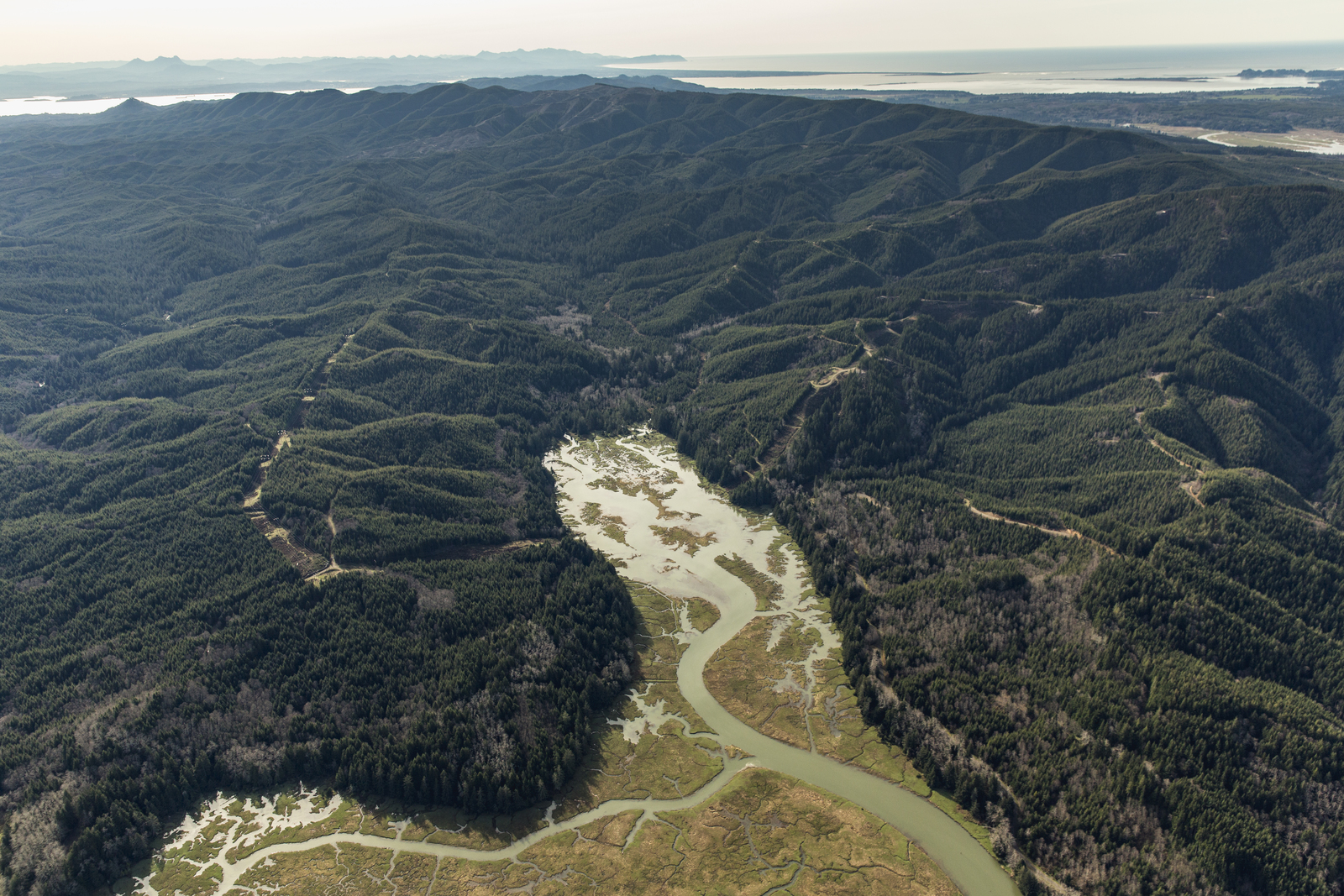An overhead aerial photograph captures a stunning, rugged mountain range blanketed in dense green trees. The landscape is intricately shaped with peaks and valleys, and subtle trails can be seen on the mountain tops. At the bottom of the image, a river meanders through the scene, flowing upwards from the bottom, snaking to the left and then turning back down, creating a complex network of waterways that diverge and converge. This river transforms into a marshy area in the middle, where water spreads into smaller rivulets between the mountain ranges, creating a swamp-like expanse. Off in the background, the faint outline of an ocean or lake is just visible, bordered by a distant, hazy line of more mountains, enhancing the depth and scale of the terrain. The photograph is rich with natural colors, featuring vibrant greens, earthy browns, and contrasting blue and white hues, bringing the untamed beauty of this mountainous river valley to life.